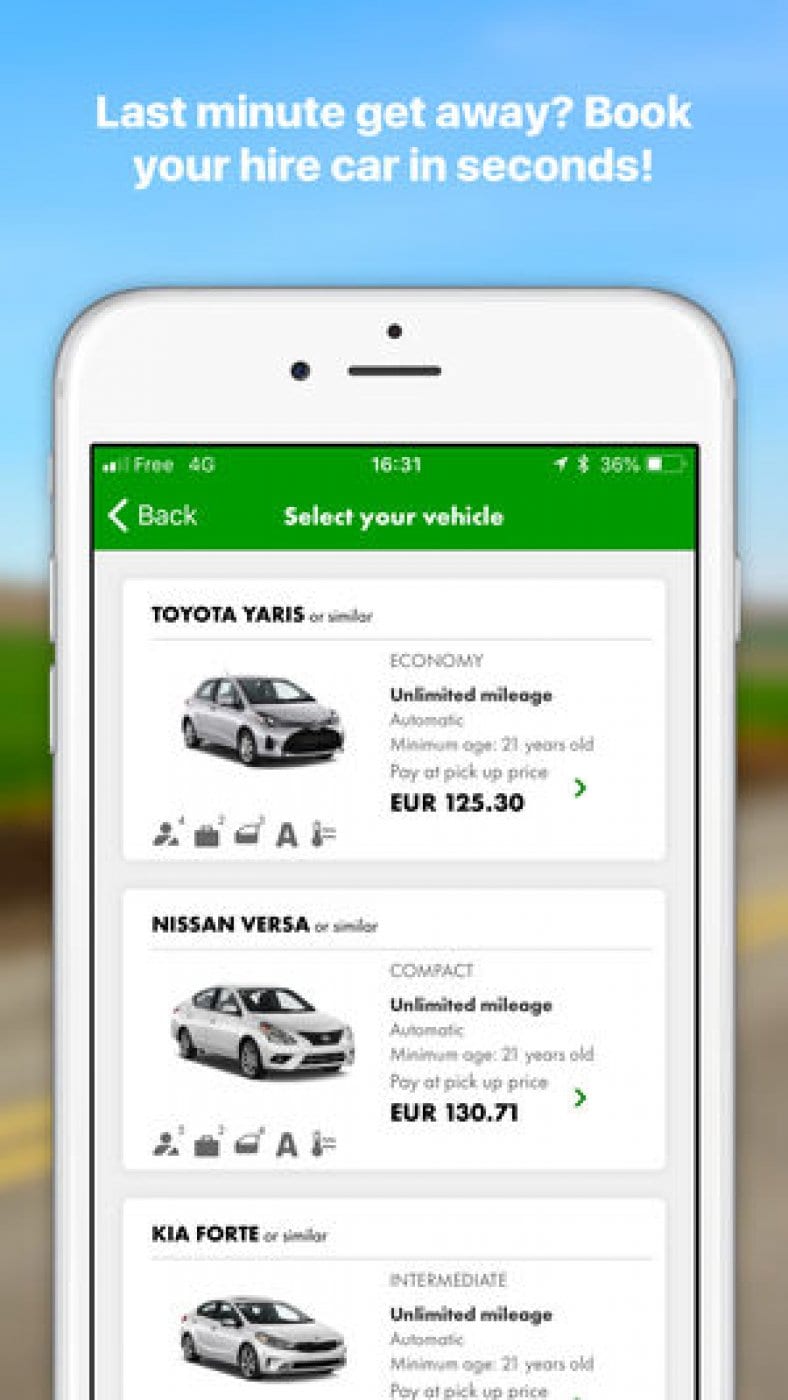This visually engaging advert for a car hire company prominently features the message "Last-Minute Getaway" in bold white text at the top of the screen. Below this headline is a close-up of an iPhone displaying the company's user-friendly app interface. The app screen includes a green banner with the text "Select Your Vehicle" in white, alongside a back button in the top-left corner for easy navigation. 

The app screen showcases three car options in white rectangles:

1. **Toyota Yaris** - Priced at €125.30, it is listed as an economy vehicle with unlimited mileage.
2. **Nissan Versa or Similar** - Priced at $130.71, it is categorized as a compact car offering unlimited mileage.
3. **Kia Forte** - This intermediate car option also offers unlimited mileage, but its full price is partially cut off at the bottom of the screen.

The cars depicted are in light, silvery, or white colors, adding a sleek and modern feel to the advert, enticing viewers with the ease and accessibility of booking a last-minute vehicle through their mobile app.